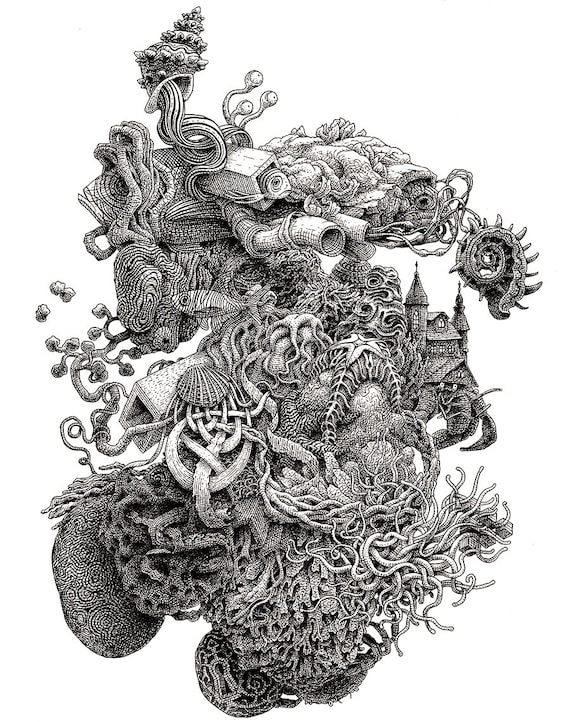This black and white pencil sketch is a detailed and elaborate depiction of a surreal, oceanic scene. At first glance, it presents an intricate cluster of various coral types and other sea elements, such as brain coral, starfish, anemones, and seashells. The central mass, which vaguely resembles a human heart in its asymmetrical blob shape, is teeming with underwater life. Among the natural coral formations, there are also mystical and bizarre elements, including braided botanical ribbons and tubes, some of which feature human-like eyes. The sketch is highly detailed, revealing small, whimsical details such as a tiny castle perched on a crab's back on the right-hand side. In the midst of the dense coral, there are also hidden creatures — a fish peeks out from between the plant life at the top, another hides in a hollowed-out brick, and peculiar long, spindly appendages emerge from a shell at the very top. This imaginative drawing, set against a stark white background with no other objects, captures a fantastical underwater world, intricately meshed together into a single, otherworldly composition.